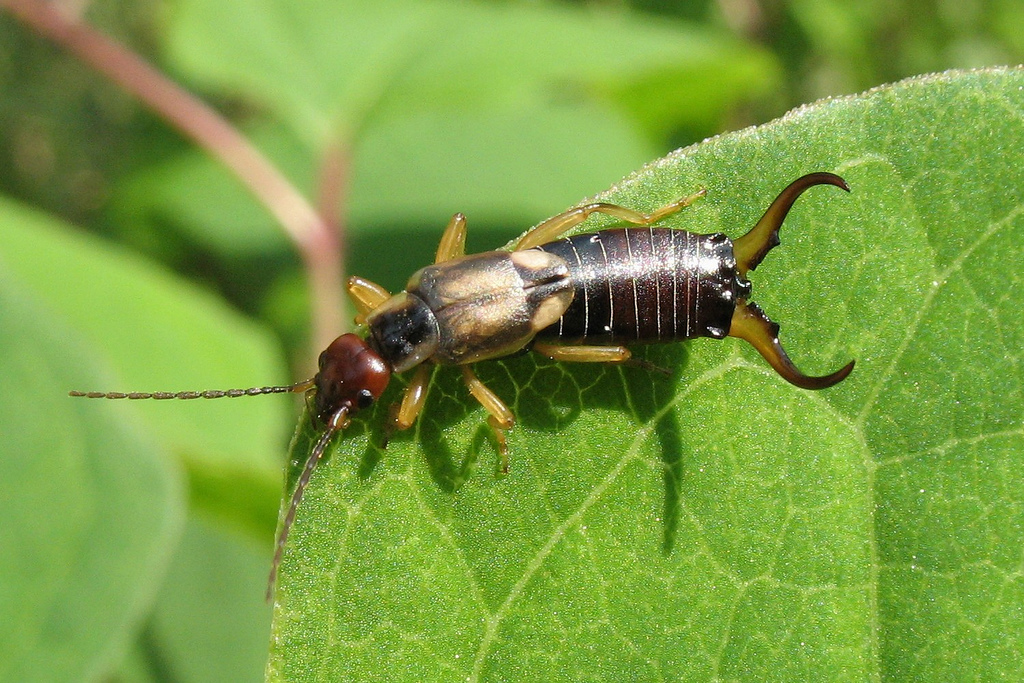In this detailed close-up photograph taken outdoors, a bug, likely an earwig, is poised on a large green leaf. The earwig's body showcases a mix of dark and light browns, with a pronounced feature of large pinchers or mandibles projecting from the end of its thorax. Its head is brown and equipped with two antennae extending to the left and right, alongside visible black eyes, one of which is more prominent than the other. The insect's six legs display a pale orange or light brown hue. Behind this sharply focused earwig and leaf, the background transitions into a soft blur, hinting at additional foliage and leaves without drawing attention away from the main subject: the earwig situated on the leaf.